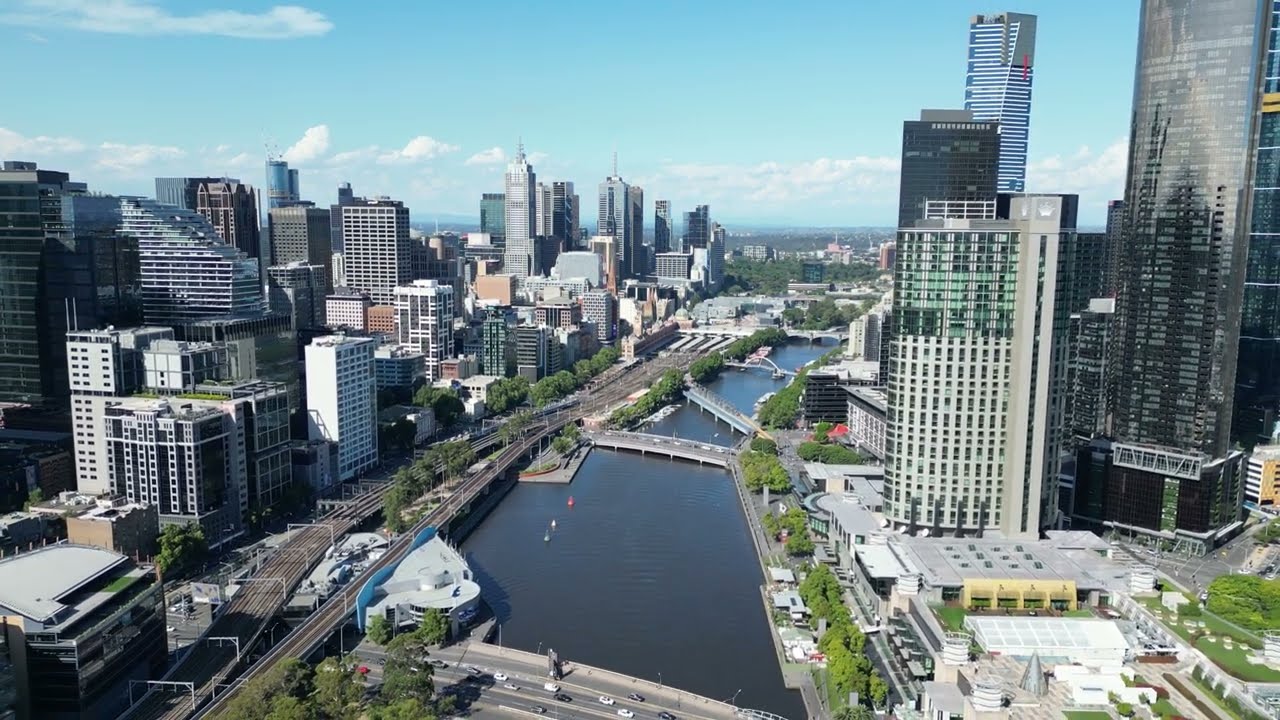This image is a color landscape photograph, taken from above using a drone, capturing a vibrant urban scene likely in either Minnesota or Chicago. Dominating the center of the image is a river with clear aqua blue waters, flanked by an array of bridges that crisscross this central waterway. To the left of the river, the cityscape is denser with high-rise buildings and skyscrapers, giving it a bustling, urban feel. A major highway runs alongside, adding to the commercial vibe of this section. In contrast, the right side of the river hosts slightly fewer buildings, including high-rises and residential structures, with more greenery interspersed. Toward the front of this side, parking decks are visible. Multiple cars can be seen on the roads, and various small boats navigate the river. The sky above is a clear blue adorned with puffy white clouds, capturing a bright, midday ambiance. The photograph showcases a realistic portrayal of urban life with a detailed representation of colors including blue, white, gray, brown, yellow, orange, pink, and green.